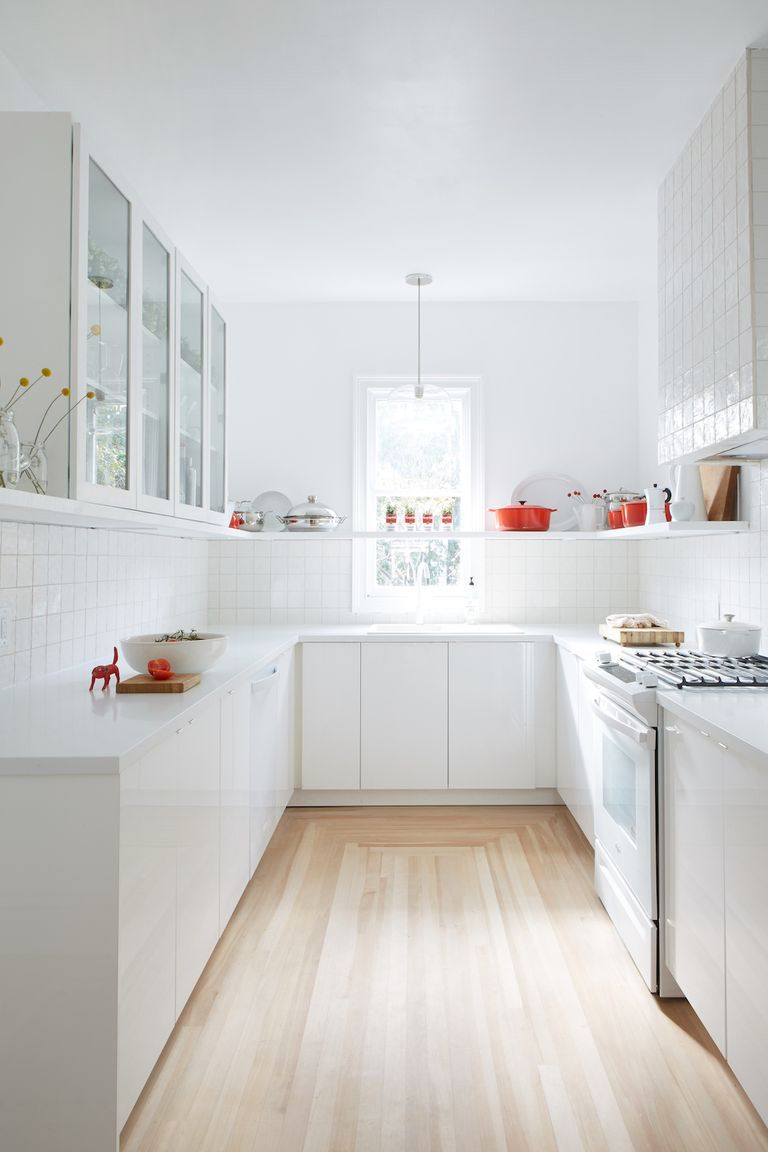The photo showcases a bright, white-painted kitchen. The space features light brown hardwood floors with darker lines and grooves. Along the left, right, and back walls, there are white cabinets with a mix of glass inserts and solid fronts. The countertops are either granite or marble in a white hue, with a running white tile backsplash connecting the countertops and cabinets.

The right side of the kitchen features a predominantly white stove with a black or gray top, upon which sits a white crock-pot. Adjacent cabinets are accompanied by a vent hood above. On the counter, there are white dishes, including bowls and plates, as well as a couple of cutting boards. One brown stick-style cutting board with legs holds a sliced tomato, bathed in sunlight streaming through a window on the back wall.

The backsplash between the countertops and cabinets displays a selection of kitchenware, including red pots, silver platters, white plates, and clear measuring cups. A grouping of four red flower pots, sprouting green plants, adds a pop of color to the space, positioned on the windowsill. A light fixture with a circular design hangs from a white cord above the window, casting illumination over this cozy culinary area.